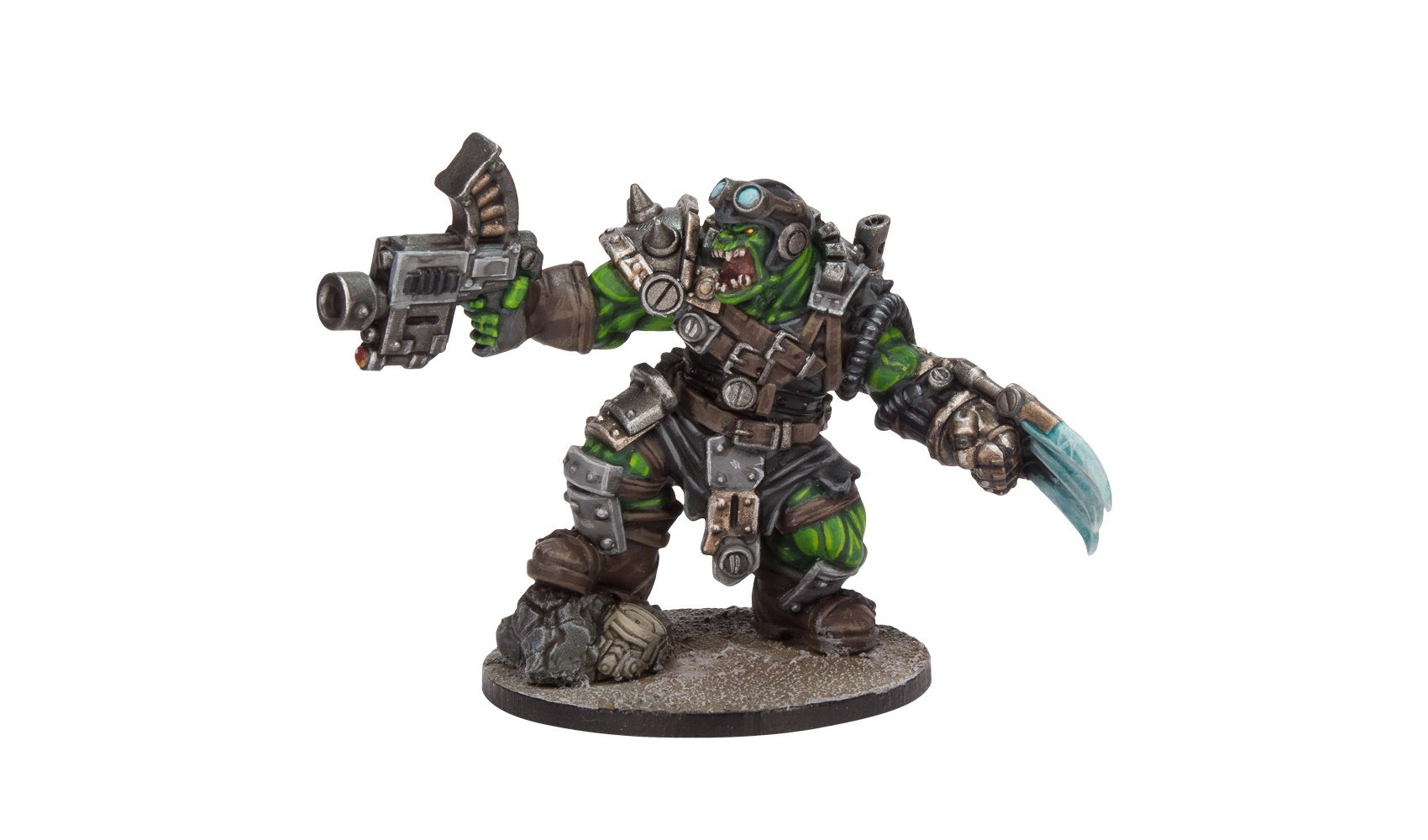The photograph in front of me depicts a highly detailed figurine set against a white background. The character is a green, reptilian, science-fiction figure, possibly a goblin or lizard-like creature, covered in an extensive array of armor. The armor includes a chest plate, shoulder pads, knee pads, a metal belt with various metallic objects hanging from it, and massive boots. The figure is adorned with leather gloves, a helmet, and metal goggles. Numerous straps and equipment pieces are fastened across its body, rendering much of its form invisible beneath the gear.

The figurine is posed on a circular, bronze-colored base, with its right foot propped up on a rock for added dynamism. In its right hand, the character wields a formidable machine gun, loaded with ample ammunition. The left hand brandishes a sword-like weapon, possibly with a wolverine-type claw apparatus or bluish pointed object, emphasizing its combat readiness. The character faces left, pointing the gun straight ahead, creating a sense of imminent action and vigilance. Overall, the figurine conveys a fierce, battle-ready presence with its detailed, multifaceted armor and weaponry.